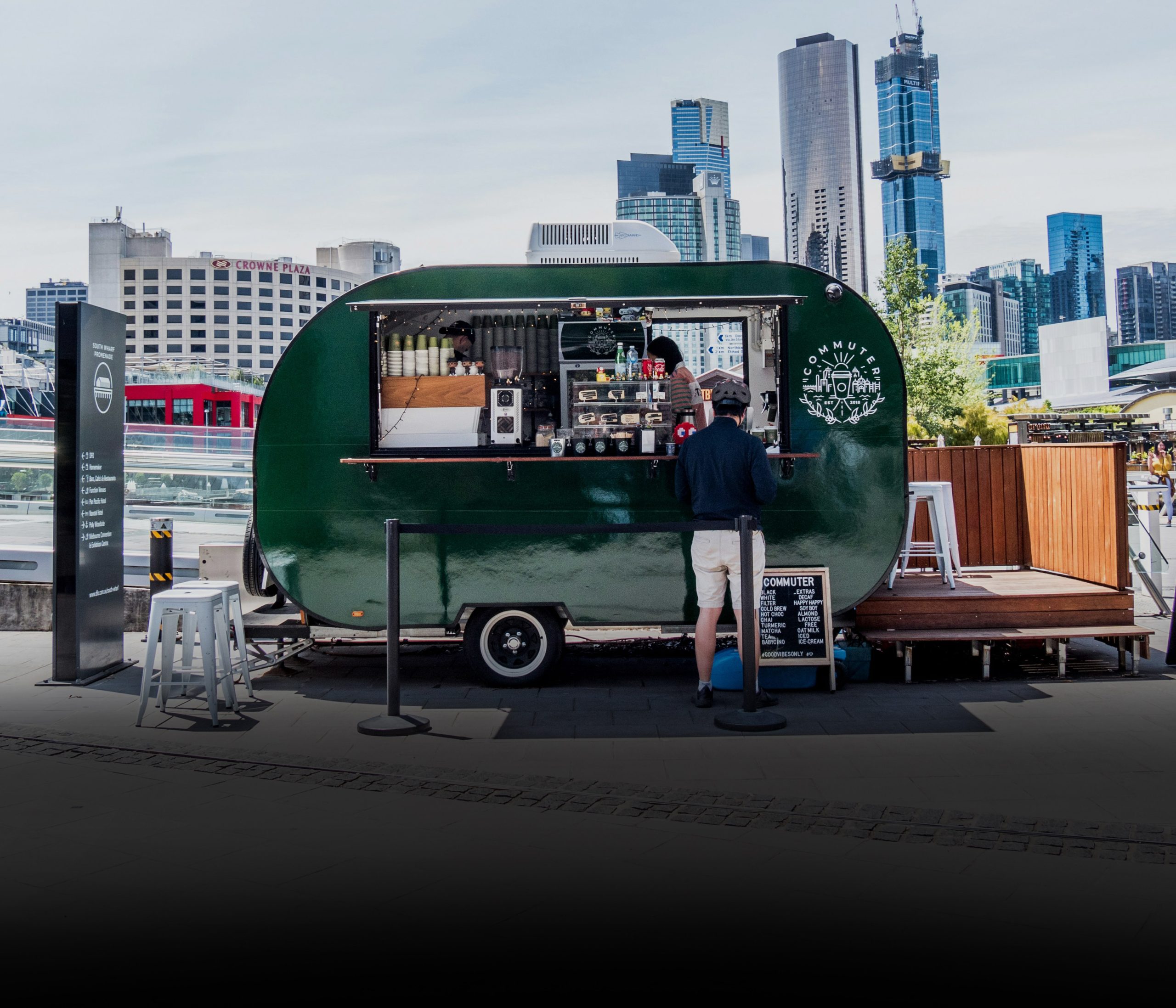This image showcases a gleaming green, round food trailer with a large serving window, showcasing various food stands inside. The interior features a prominent silver cabinet positioned centrally, and to the left, there's a wooden shelf adorned with numerous cups, suggesting a streamlined setup for beverages. A sizable coffee maker dominates the background near neatly stacked cups. A person is visible behind the window, indicative of readiness to serve, while below the window, a wooden ledge extends outward. A customer, seen from behind, waits on the asphalt lot; he's attired in beige shorts, tennis shoes, a navy blue long-sleeve shirt, and is wearing a helmet.

In the backdrop, a cityscape of towering high-rise buildings punctuates the scene. Blue skyscrapers with abundant windows stand prominently, and to the left, a large gray high-rise branded with "Crowne Plaza" in red letters is notable. The food trailer prominently displays the word "Commuter" both on its body and on a small beige wooden sign placed in front, which features a black chalkboard section with white lettering, albeit mostly unreadable. An awning extends from the trailer's top, beneath which an air conditioning unit is visible.

A little wooden deck with white stools is situated to the right of the trailer, basking in sunlight, while further left, additional white plastic stools are scattered. Behind this setup, there’s a semi-transparent white fence and a red structure whose purpose is unclear - potentially another building or a marina. A sturdy dark brown metal sign affixed to the parking lot adds another layer of detail, though its white inscription remains unreadable.

The entire scene is set in a black asphalt parking lot, with bright sunlight casting a welcoming hue over the whole area.